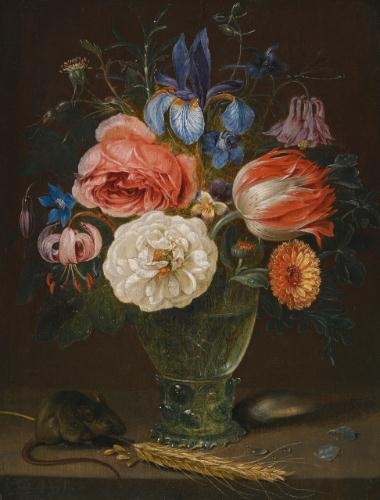The image showcases an exquisite bouquet of flowers in a clear glass vase, filled with water up to about 80% of its capacity. The bouquet boasts a rich array of colors including a prominent yellow sunflower, a pink rose, blue flowers, a striking large white flower in full bloom, and other blooms in shades of orange and white. Notably, a purple flower droops to the right, and a bulb-shaped flower leans towards the bottom. Set against a dark, yet not overly somber background, this vibrant display of nature is complemented by a small brown mouse. The mouse is nibbling on what appears to be a piece of grain or wheat lying flat on the table beside the vase. The overall setting lends a harmonious blend of natural beauty and delicate still-life composition.